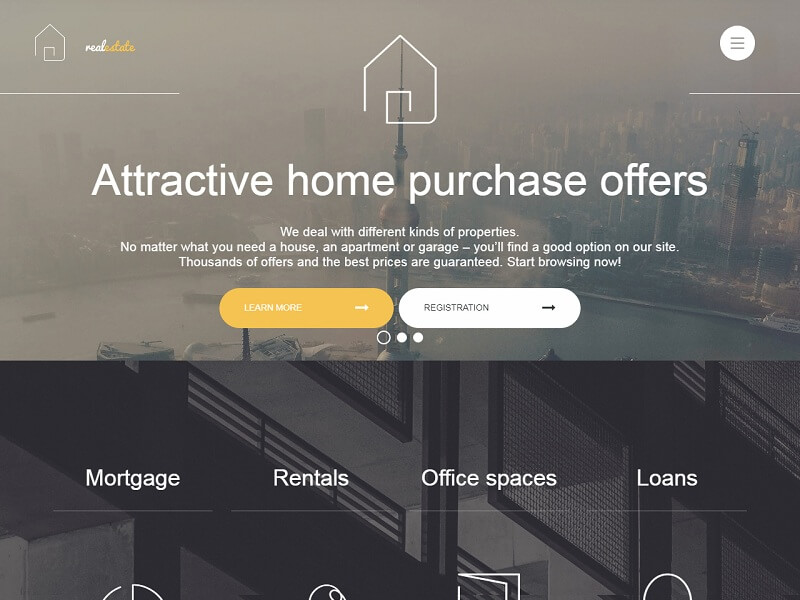Screenshot of a Website Offering Home Purchase Deals

The webpage is titled "Attractive Home Purchase Offers," prominently displayed at the top center of the screen with a larger home icon situated above it. In the upper right corner of the page, a white hamburger menu provides easy navigation, while a smaller home icon is positioned on the left side.

Directly beneath the main title, a subheading states: "We deal with different kinds of properties. No matter if you need a house, an apartment, or a garage, you'll find a good option on our site. Thousands of offers and the best prices are guaranteed. Start browsing now."

Below this informative text are two call-to-action buttons: a vibrant yellow "Learn More" button on the left, and a white "Registration" button on the right. Underneath these buttons, three navigational dots are displayed, with the first dot in gray and the other two in white, indicating the user's current position on the webpage.

Further down, the website is divided into four distinct sections: Mortgage, Rentals, Office Spaces, and Loans. Each section is denoted by a descriptive title along with a corresponding icon to visually represent the category. The overarching background of the webpage features a cityscape with the tops of buildings visible at the top portion and a darkened parking garage forming the lower part of the backdrop.